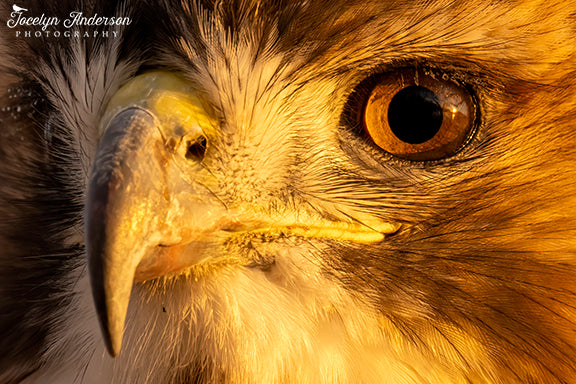This is an extremely detailed close-up photograph of a bald eagle captured by Jocelyn Anderson Photography, as indicated in the top left corner of the image. The eagle's face dominates the frame, highlighting distinct features that emphasize its predatory nature. The beak is prominently curved and pointy, with a sharp grayish front transitioning into a yellow base; it also has visible nostril openings. The eagle's eyes are intense, with a striking combination of black pupils and brown or golden irises that give it a piercing stare. Surrounding the beak and underneath it, the feathers are predominantly white, while the rest of the face features a mixture of brown and gray feathers. The eagle's serious and formidable expression is perfectly captured in this high-resolution image.